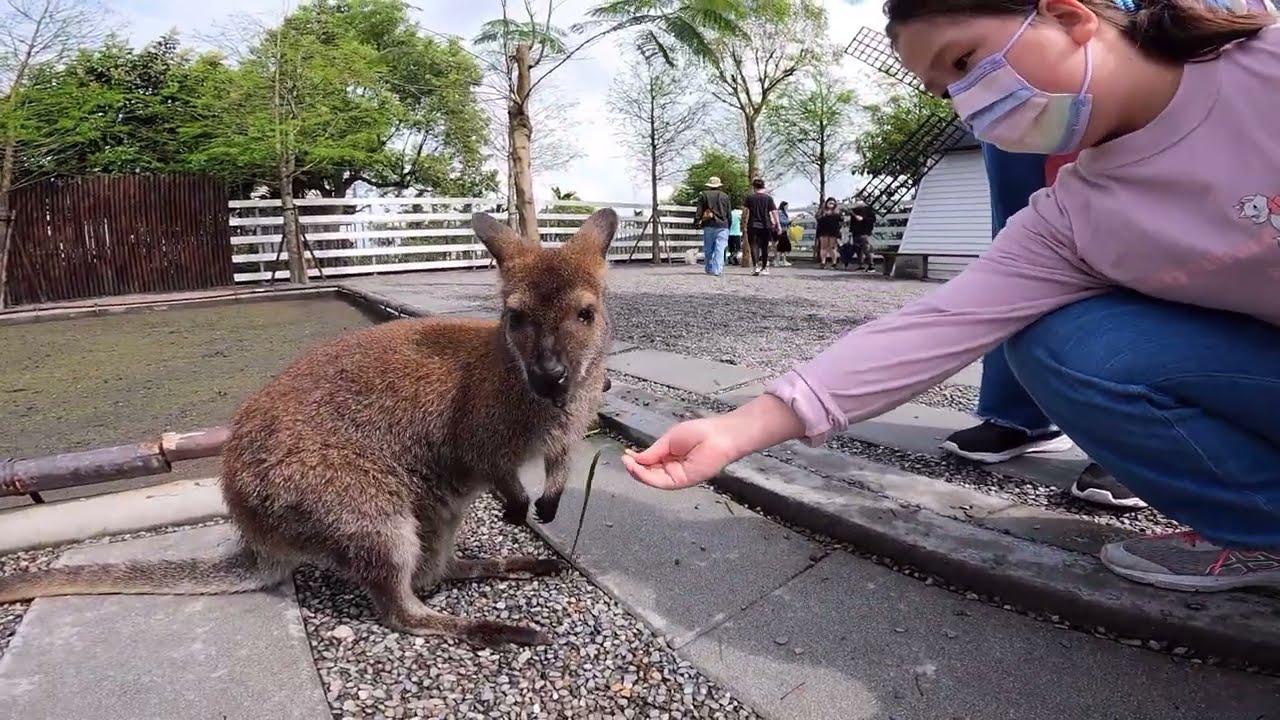In this outdoor daytime photograph, a young girl stands on the right-hand side extending her right arm towards a baby kangaroo or wallaby, which is looking directly at the camera. She is dressed in a long-sleeved pink shirt featuring Marie the Cat, blue jeans, gray sneakers, and a face mask adorned in shades of pink, blue, purple, and green. The girl and the kangaroo-like creature are positioned on gray pebbles bordered by gray paver stones. The kangaroo has a long tail, brown fur with black-tipped paws, and upright ears. In the background, a mix of blue sky, green trees, wooden fencing, and other zoo visitors can be seen. Notably, the fence transitions from long white planks to tall dark wood, and there's a stylized, non-functional windmill near the midpoint. The scene suggests a lively zoo setting with various elements of nature and human activity intermingling.